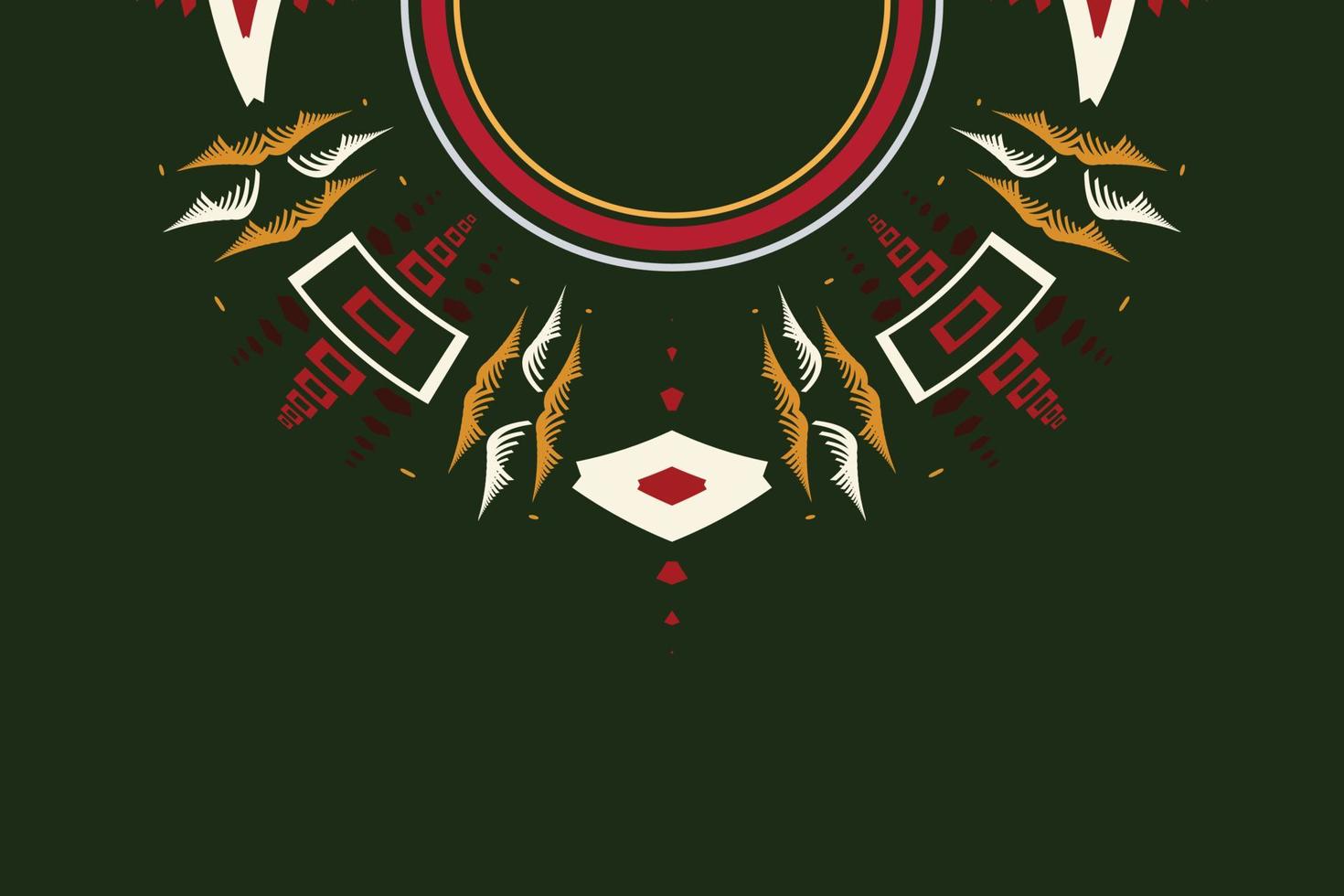The image is a digital illustration set against a dark hunter green background, possibly depicting a modern neck design. At the top center, there are three concentric half circles: the innermost being a thin yellow line, followed by a thicker red line, and an outer thin white line. These arcs are surrounded by various geometric shapes in a pattern, including squares, rectangles, and diamonds, predominantly in red and white. The shapes seem to radiate outward, resembling rays or design vectors that expand from the circles before tapering back. This structured yet intricate arrangement of yellow, red, and white colors creates a dynamic visual effect against the dark green backdrop.